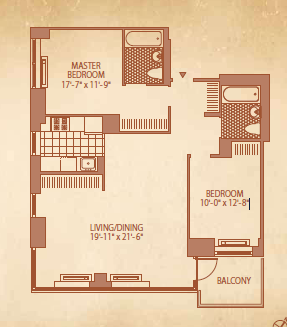The image depicts a vertically oriented rectangle with a textured gradient background, transitioning from a darker tan and beige at the top to a lighter tan and beige at the bottom. In the bottom right-hand corner, there is a small semi-circle containing a "V" shape. Dominating the image is a computer-generated blueprint of a house, rendered in brown lines against the background. The blueprint provides a flat, head-on view of the house layout.

At the top section of the blueprint, the master bedroom is labeled, along with its dimensions and an adjoining bathroom that includes a bathtub. Near the entrance of the house, there's another bathroom, also equipped with a bathtub, positioned close to the second bedroom. The central area of the blueprint details the living room and dining room spaces, and from here, one can access a balcony directly connected to these communal areas.